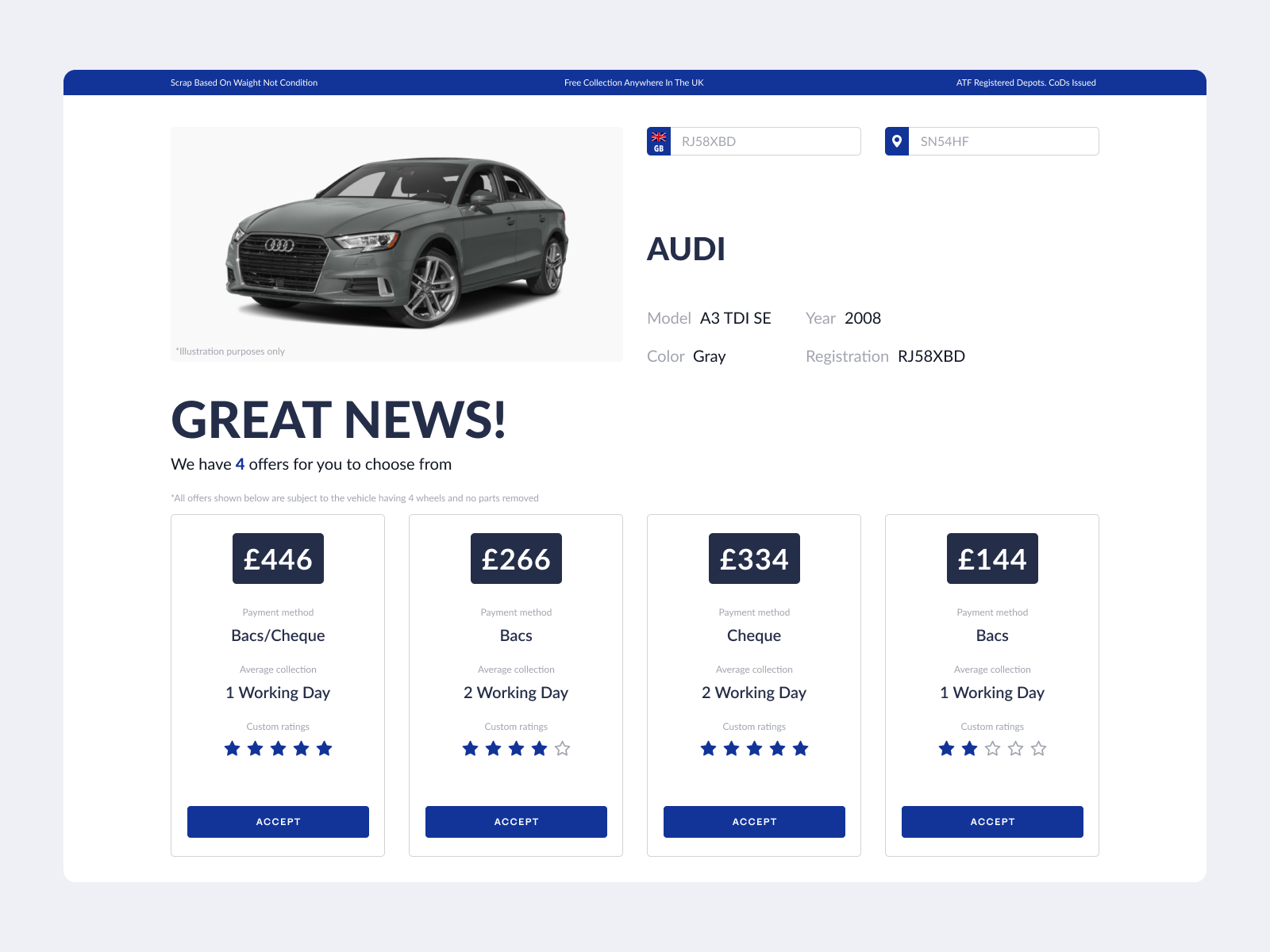This is a screenshot taken from a computer screen, featuring a user interface with a predominantly gray background. Superimposed on this background is a prominent white rectangle. Within this rectangle, in the top left-hand corner, there is an image of a gray car accompanied by the text "Audi" spelled out as A-U-D-I. Detailed specifics for the car indicate it is a 2008 model, further described with the color gray, and includes both the model number and registration number.

Below the car details, there is a message that reads, "Great news, we have four offers for you to choose from." Beneath this message, four rectangular boxes are arranged towards the bottom of the picture, each displaying an offer with a price listed in pounds. The first offer is for £446, the second for £266, the third for £334, and the last for £144. Each box also specifies the payment method as "backs or check," the number of working days required—typically between one or two days—and a star rating for each option.

At the bottom of each of these boxes, there is a clickable blue area labeled "Accept," allowing the user to select their preferred offer.